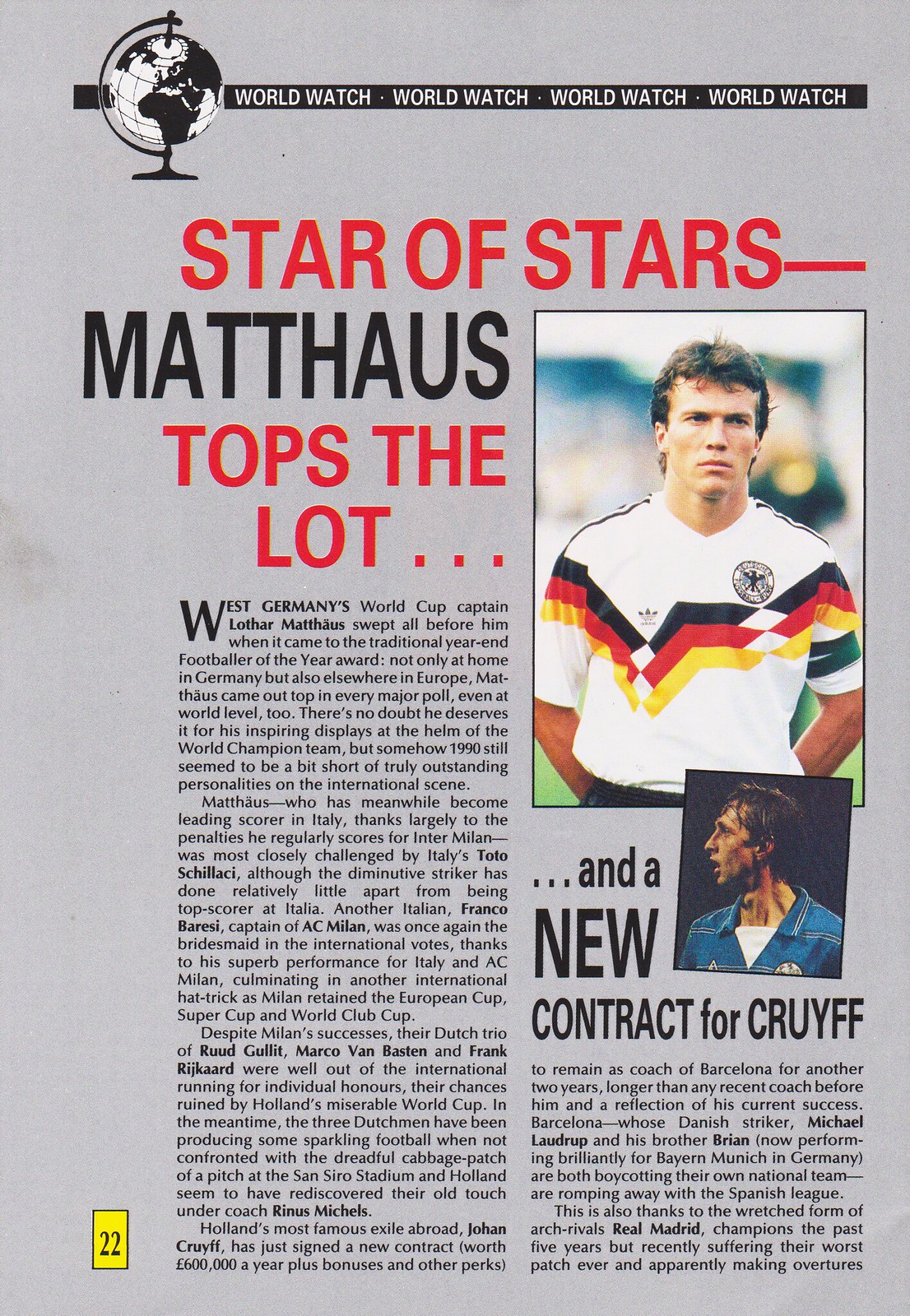The article features a detailed layout showcasing a prominent soccer player, highlighting his exceptional achievements. At the very top left, a black and white globe is depicted, symbolizing the global theme of the publication, with the words "WORLD WATCH" repetitively positioned within a black rectangle. This suggests that the magazine could be named "World Watch." Dominating the header in striking red and black text, the title reads "STAR OF STARS" with "Matthaus" in bold black, followed by the phrase "tops the lot" in red. 

To the right of the title, a picture of the soccer star, presumably Lothar Matthaus, is featured. He is seen in the iconic white West German soccer jersey, adorned with jagged black, red, and yellow stripes along with the German eagle emblem, indicating his identity as the World Cup captain for West Germany. Below this, a smaller mention hints at another article involving a contract for the renowned player Cruyff.

The main section comprises an extensive article, spanning several paragraphs, detailing Matthaus’s career and his pivotal role in leading West Germany in the World Cup. Additionally, a distinctive small yellow rectangle marked with the number 22 is located at the bottom left, potentially indicating a page number or specific detail related to the article.